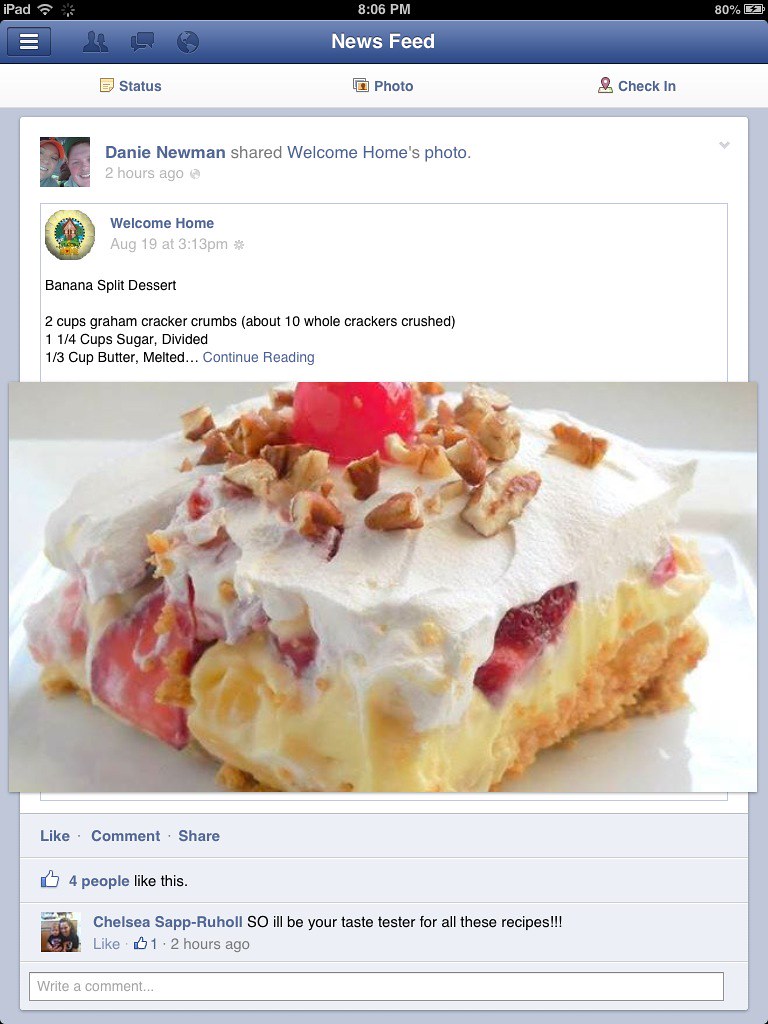This is a screenshot from an iPad displaying a Facebook News Feed at 8:06 PM with 80% battery life. At the top left, the iPad label and Wi-Fi signal icon are visible. The Facebook interface shows the News Feed banner with icons for notifications and messaging. Danny Newman shared a post from "Welcome Home" that was originally posted on August 19th at 3:13 PM, featuring a banana split dessert recipe. The dessert is a square-shaped slice with a graham cracker crust, a custard-like pudding layer, a layer of whipped cream topped with strawberries, chopped walnuts, and a cherry. The post includes options to Like, Comment, and Share; it has four likes and one comment from Chelsea Sapp-Ruhol, who humorously offers to be the taste tester for the recipes. Her profile picture is displayed beside her comment, and underneath it, there's a write comment box for additional interaction.